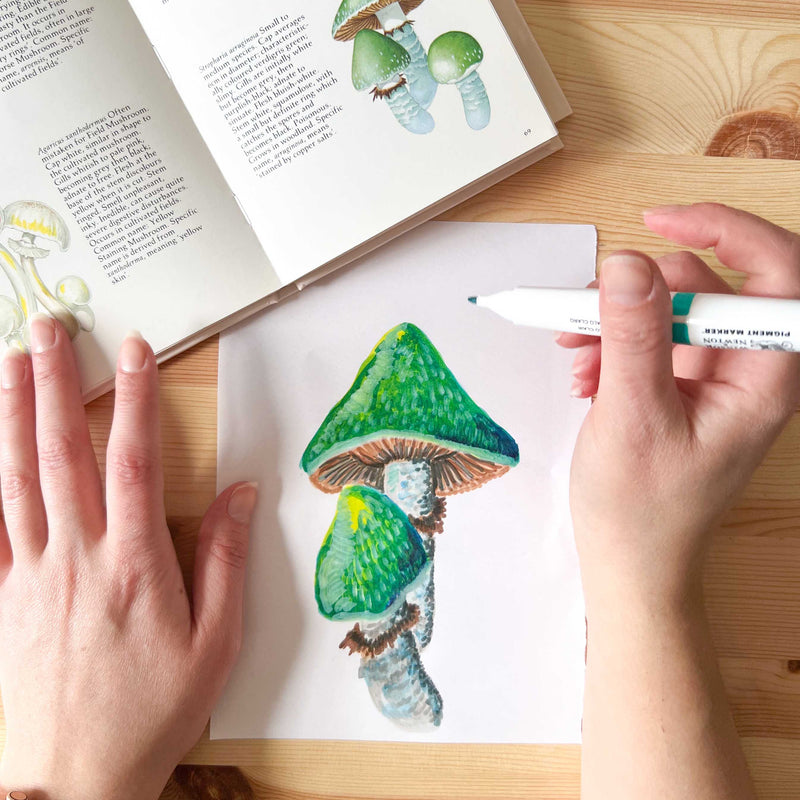In the photograph, a young artist sits at a light brown wooden desk, diligently painting a detailed illustration of vibrant green mushrooms with white stalks and orangish gills. The child's small hands are clearly visible, their right hand grasping a white pen as they bring the whimsical fungus to life on a clean sheet of white paper. At the top left of the image, an open book rests on the desk, its white pages adorned with black text and illustrations of mushrooms, seemingly guiding the child's artwork. The desk's wood grain texture adds a warm backdrop to the creative scene, emphasizing the artful and studious atmosphere.